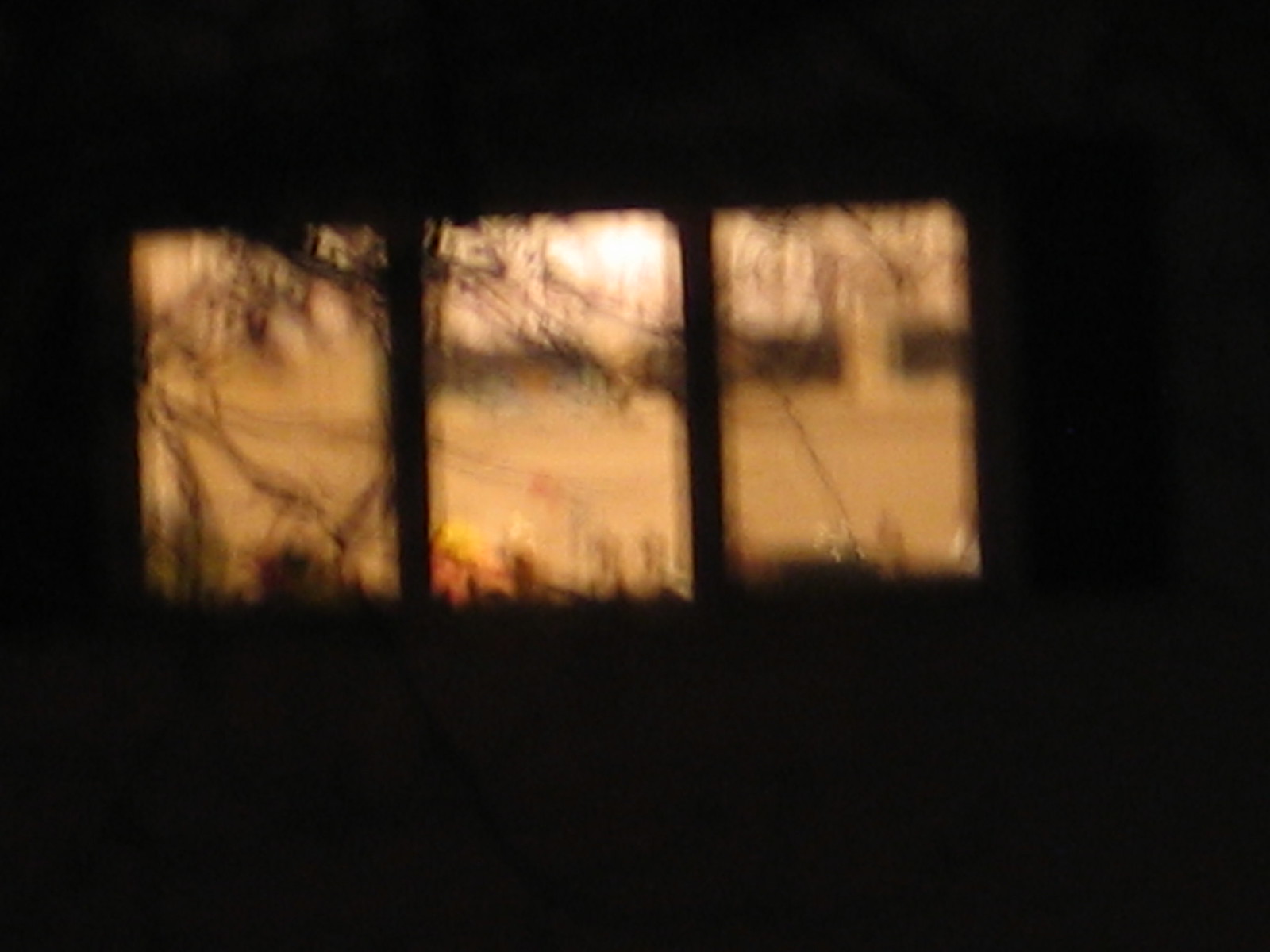This is a somewhat blurry photograph capturing a distant view of a three-paneled window. The window is partially obscured by tree branches both in front of and visible through it. At the base of the window, there are faint hints of orange coloration. The left side of the scene features some yellow tones, while pale green hues subtly emerge in the surrounding area. The ground outside the window appears to be a tan color, interspersed with patches of grass. Additional trees populate the background, through which the Sun can be seen shining, casting a hazy light that contributes to the overall blurred quality of the image. The right side of the image is predominantly dark, making it difficult to discern further details amidst the shadows and blurred elements.